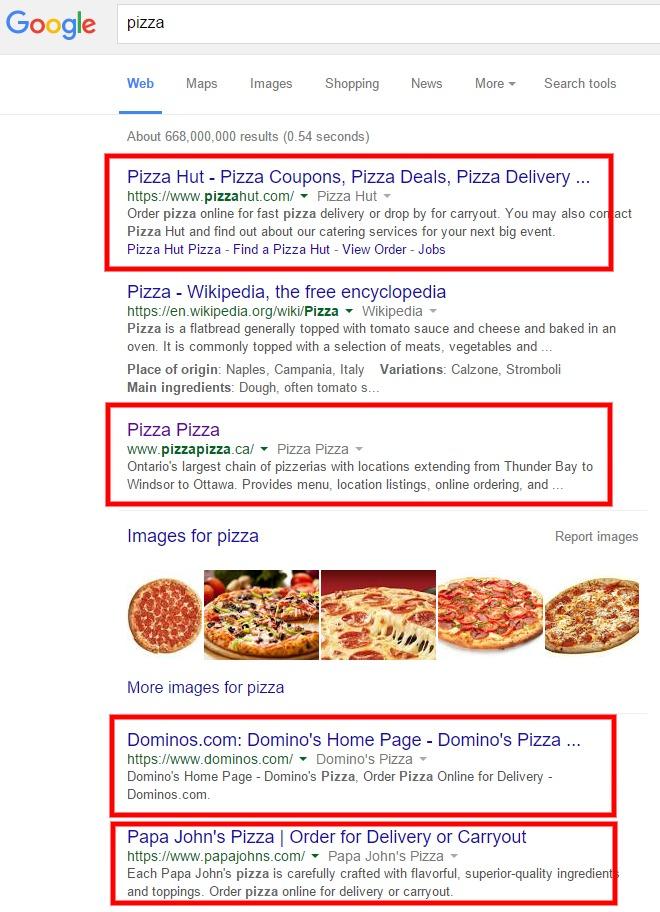This section displays a Google web search for "pizza." The initial result highlights a web search category, followed by links including Pizza Hut, Pizza Coupons, Pizza Deals, and Pizza Deliveries. Beneath these, there is a link to the Wikipedia page for pizza, labeled "Pizza - Wikipedia, the free encyclopedia." The subsequent result is a link to a site labeled "Pizza Pizza" with the URL www.pizzapizza. Below these text-based results, there is a horizontal array consisting of eight images of various pizzas. The images feature a variety of toppings including pepperoni and cheese, olives, extra cheese, and combinations thereof, such as double cheese and pepperoni. Users have the option to click on these images to view more pizza-related visuals.